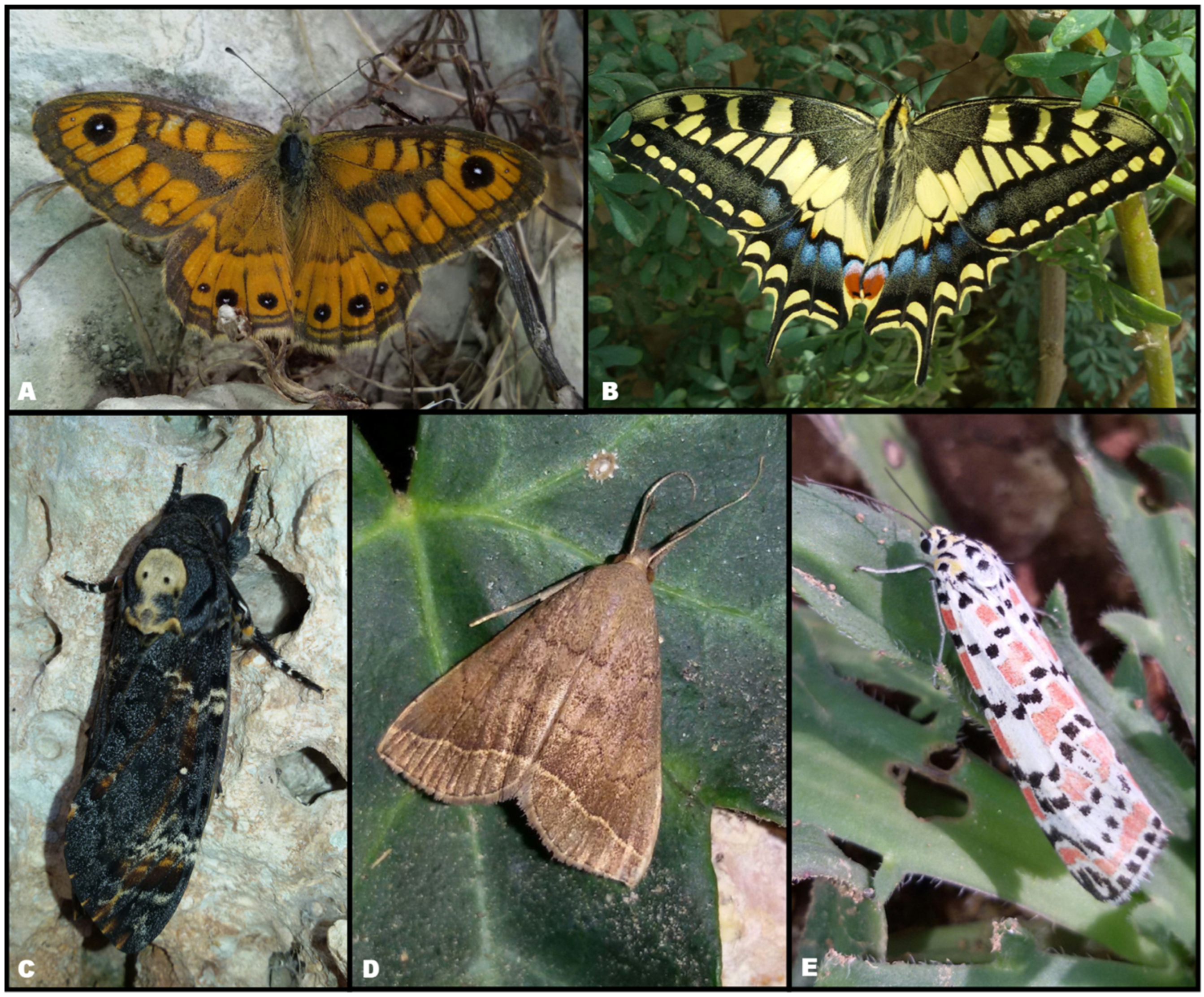This image is a detailed collage consisting of five different colored photographs of insects, each labeled from A to E. 

Letter A, positioned in the top left, shows an orange and brown moth with its wings spread out. The wings are adorned with black spots, each containing a white dot inside. 

To its right, labeled as B, is a yellow butterfly with highly pointed wings, featuring an orange hue near the bottom center.

The image labeled C, located in the bottom row, depicts a moth with a long black body and a light brown spot at the top.

Next, the photograph labeled D presents a brown moth resting on a vibrant green leaf.

Finally, the image labeled E shows an orange, black, and white moth on a leaf scarred by brown spots where it has been feeding.

Overall, the collage portrays a variety of both moths and butterflies, showcasing their diverse wing patterns and colors in a detailed and organized manner.